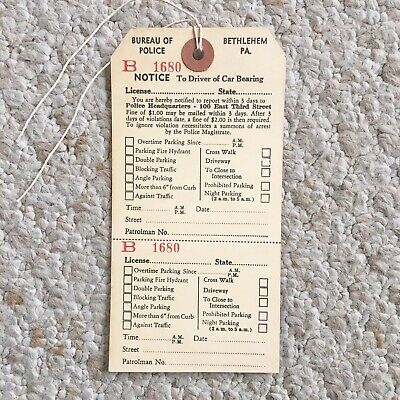This photograph features a manila-colored vintage police tag, resembling an old parking ticket, placed on an off-white carpet with beige spots and a woven texture. The tag, possibly an amateur photograph, has a circular hole reinforced by a keeper with a white string attached. At the top left, it reads "Bureau of Police," and on the top right, "Bethlehem PA," followed by a burgundy serial number "B-1680." The text continues in black, stating, "Notice to Driver of Car Bearing," with dotted lines for "License" and "State." It instructs the driver to report within three days to police headquarters at "100 East 3rd Street," highlighting a fine structure: $1 if paid within three days, and $2 thereafter. Non-compliance may lead to arrest. The tag includes various checkboxes for infractions such as overnight parking, parking near fire hydrants, double parking, blocking traffic, and more. The same information is repeated on the lower part of the tag, designed to be torn off.